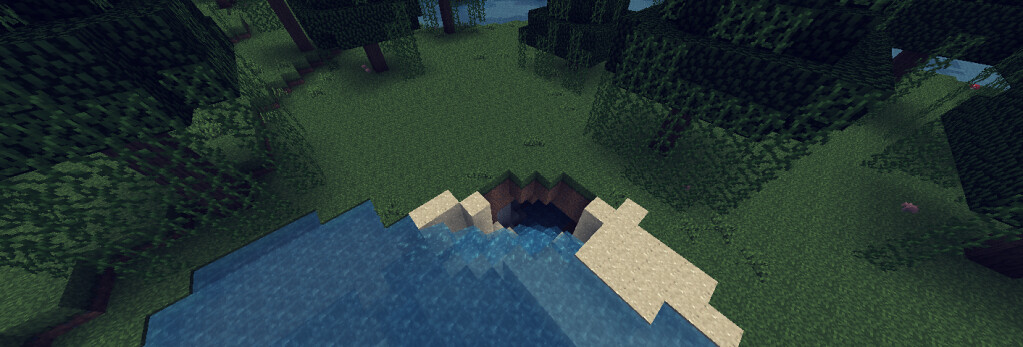The image appears to be a top-down view of a computer-generated scene, reminiscent of a Minecraft environment with its blocky aesthetic. The scene is a complex, multi-colored landscape featuring various shades of green, representing trees and vine-like foliage hanging vertically. At the forefront, there is a blue, blocky structure that could resemble a hot tub or a small pool, bordered by white blocks. The scene includes several brown structures and a brown hole in the ground. Additionally, there are blue areas both at the top and to the right side of the image, perhaps indicating water bodies like a lake or river. Pink elements are scattered on the right side. The overall view is both intricate and confusing with its mix of colors and blocky forms, making it appear like a digitally rendered or a Lego-like creation.